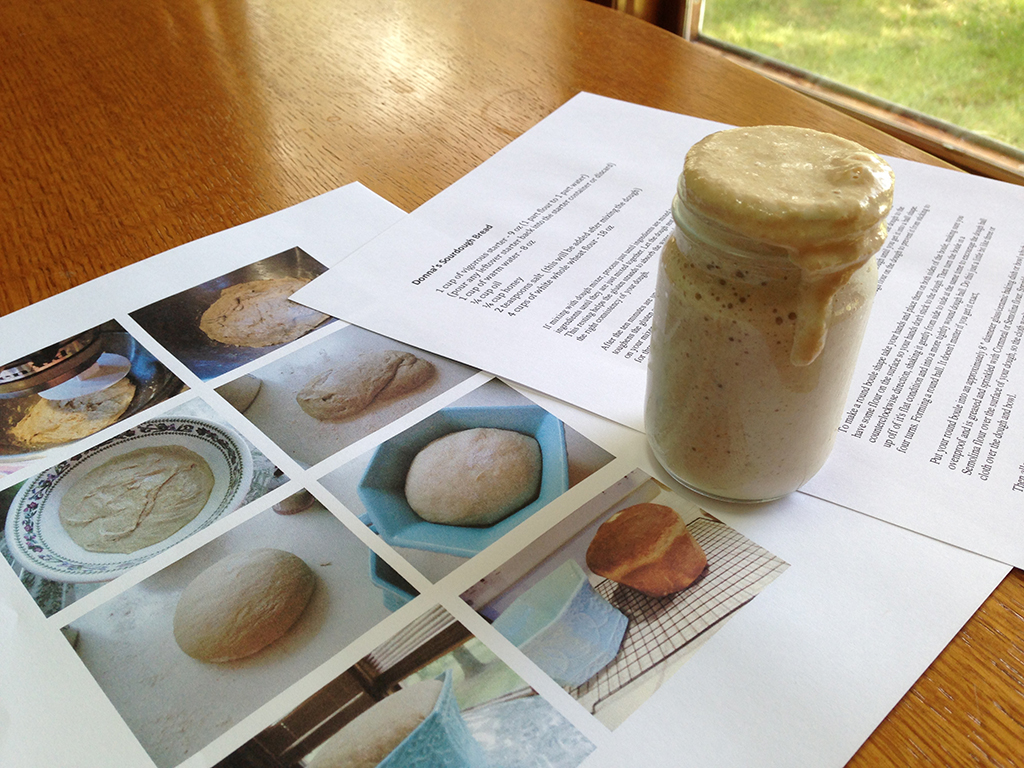The image depicts a brown wooden dining or kitchen table with two pieces of paper laid out on top. On the left piece of paper, there are eight images showcasing the step-by-step process of preparing sourdough, from initial mixing to the final baked product. The right piece of paper features the title "Donna's Sourdough Bread" in bold at the top, followed by a list of ingredients and detailed paragraphs of instructions below. On top of these papers sits a glass mason jar filled with frothy, overflowing yeast or sourdough starter, with bubbles and a tan, sandy hue. The jar has no lid, and the mixture is visibly running down its side. In the background, a window offers a view of a grassy yard, adding a sense of homeliness to the scene.